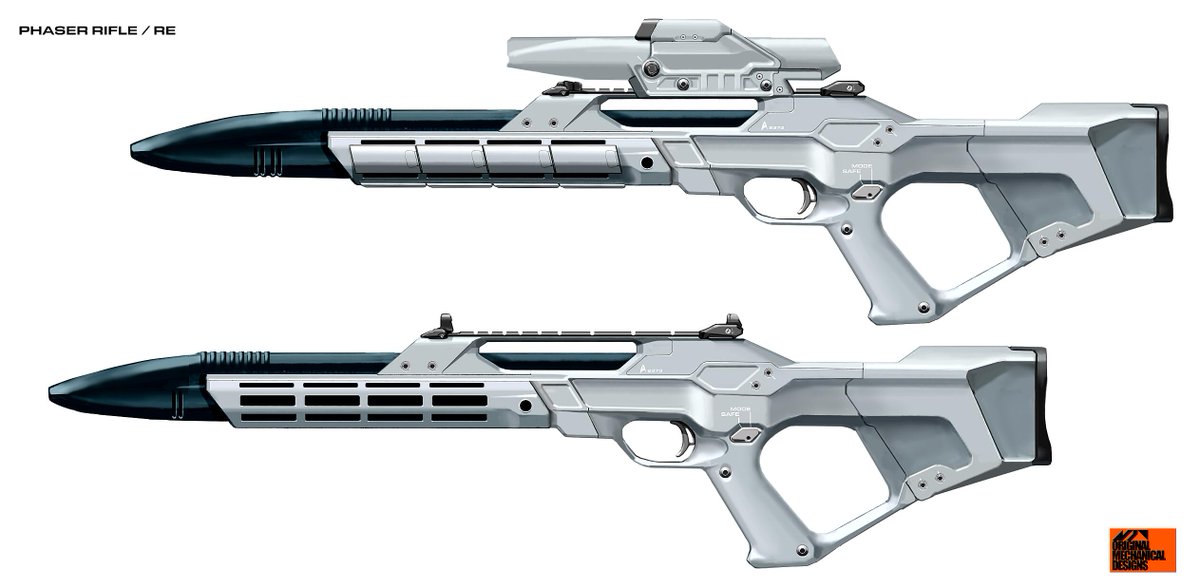This is a detailed, color photograph of two futuristic, sci-fi rifles that appear hyper-realistic, resembling something out of a Star Trek episode or a sci-fi movie rather than conventional firearms. The image focuses on the profile shots of these two rifles, both facing left, displayed against a plain white background. In the upper left corner, there is a label in black text reading "phaser rifle / RE," indicating their phaser rifle model.

The rifles, primarily silver with black details, are not identical but share many similarities. Both guns feature black, pointed barrels, typical in appearance to where bullets or other projectiles would exit. The rifle on the top is equipped with an optical sight, enhancing its futuristic look, whereas the bottom rifle lacks this feature but has a shorter stock and a mounting rack. Additionally, each rifle includes a clearly visible trigger and pistol grip, reinforcing the idea that these are highly specialized, likely collector's items, designed to stand out with their unconventional, imaginative design rather than for practical use. In the bottom right-hand corner, there is an orange box with black text, though it is too small to decipher any meaningful details from at this resolution.